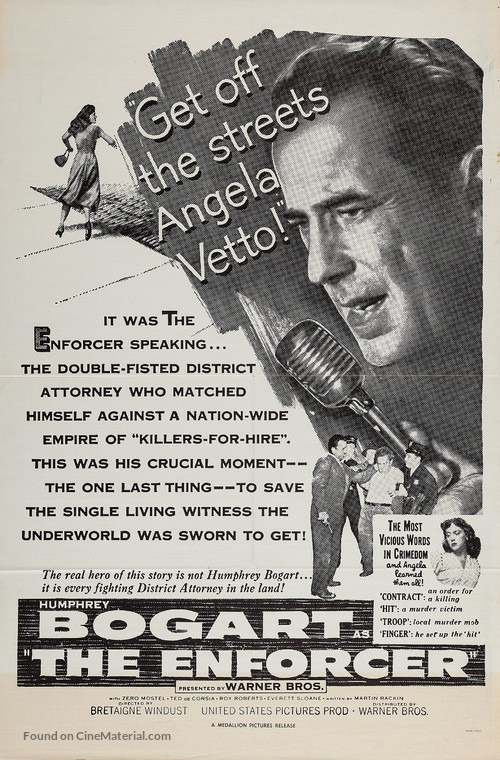This vintage movie poster from the 1940s or 1950s, printed on light beige, creme paper with black ink, advertises the film "The Enforcer" starring Humphrey Bogart, presented by Warner Brothers. The main text declares, in bold black lettering, "The Enforcer speaking, the double-fisted district attorney who matched himself against a nationwide empire of killers for hire. This was his crucial moment, the one last thing to save the single living witness the underworld was sworn to get." At the top, the phrase "Get off the streets, Angela Vetto" appears prominently. On the top right, a man with slicked-back hair, approximately 40 years old, stands in front of a microphone, seemingly delivering "the most vicious words in crimedom." A smaller image of a woman dressed in a street outfit, holding a purse, is positioned above him. The bottom of the poster features additional details and proclaims, "Humphrey Bogart as The Enforcer." An important note at the bottom states, "The real hero of this story is not Humphrey Bogart; it is every fighting district attorney in the land."